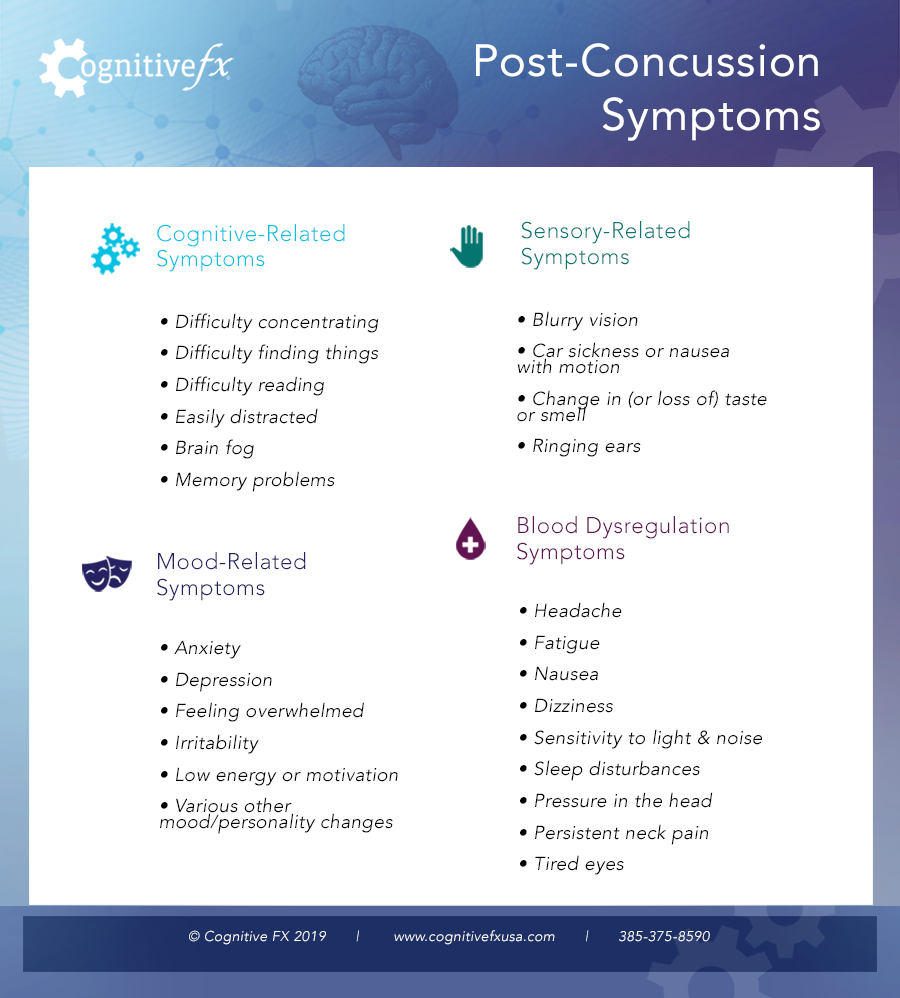The image is a detailed reference page on post-concussion symptoms from Cognitive FX, set against a gradient background transitioning from pale blue in the top left to purple in the top right. At the top left, there is a white logo for Cognitive FX, where the "C" is shaped like a gear. To the right, there is a silhouette of a human brain facing left, and above it, white text reads "Post-Concussion Symptoms." 

In the center, a large white box is divided into four sections, each with a distinct header and icon. The top left section, under a blue header with three small cog images, lists "Cognitive Related Symptoms" such as difficulty concentrating, difficulty finding things, difficulty reading, being easily distracted, brain fog, and memory problems. 

Below, the section titled "Mood Related Symptoms" is marked by a purple header with a happy and sad face mask icon. The symptoms listed here include anxiety, depression, feeling overwhelmed, irritability, low energy or motivation, and various other mood and personality changes.

To the right, the "Sensory Related Symptoms" section, denoted with green text and a hand icon, includes symptoms such as blurry vision, car sickness or nausea with motion, changes in or loss of taste or smell, and ringing in the ears.

The bottom right section, with a red header and a blood droplet icon featuring a white plus sign, outlines "Blood Dysregulation Symptoms" such as headache, fatigue, nausea, dizziness, sensitivity to light and noise, sleep disturbances, pressure in the head, persistent neck pain, and tired eyes.

At the bottom of the image, a blue rectangle contains white text with the information: "Cognitive FX 2019 www.cognitivefxusa.com 385-375-8590."